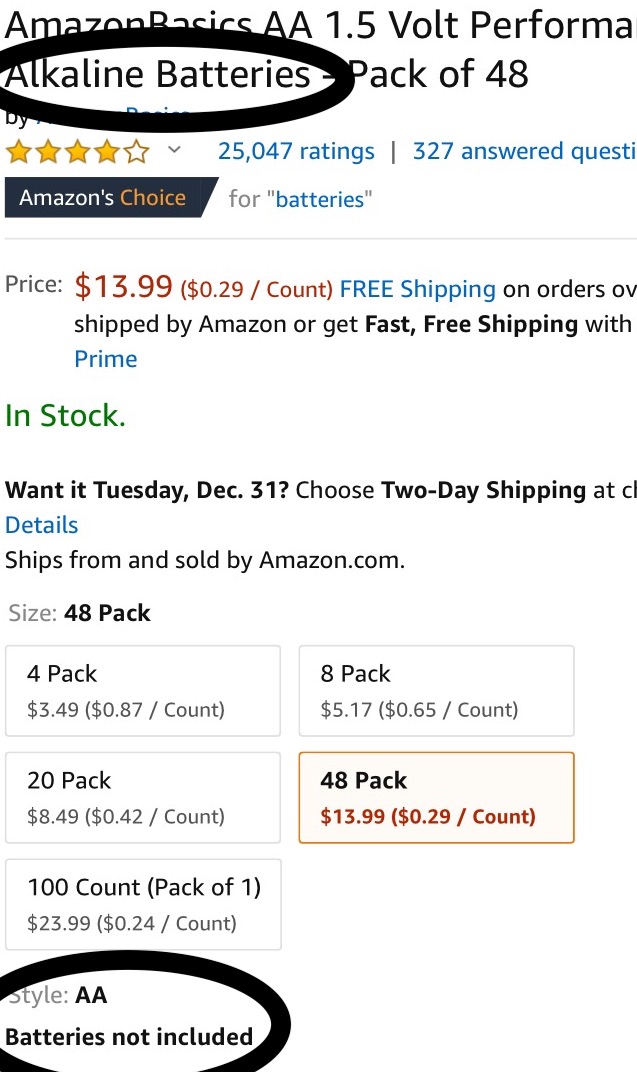This image is a screenshot from an Amazon product page, specifically formatted to look similar to a mobile phone view. It appears to be a close-up segment from a larger image, focusing on particular details for emphasis.

The screenshot highlights two main elements using black circular discs. The first highlighted text at the top reads "Alkaline batteries," while the second highlighted text at the bottom states "Style: Double-A batteries not included."

The rest of the screenshot displays typical features of an Amazon product page. At the top, "Amazon Basics AA 1.5 Volt Performance Alkaline Batteries - Pack of 48" is prominently displayed against a white background. Below the product title, the item has received a rating of 4 out of 5 stars, based on 25,000 customer ratings. The product is listed as in stock with a price of $13.99.

Additionally, the screenshot shows various quantity options available for purchase, including packs of 4, 8, 20, 48, and 100. The 48-pack option is visually emphasized with an orangish tint, whereas the other options are simply displayed in black and white. This indicates that the user has selected the 48-pack option.

Overall, the screenshot was created to draw attention to the specific details of "Alkaline batteries" and the note that "Style: Double-A batteries not included," while also providing a clear view of the product's main information and purchasing options.